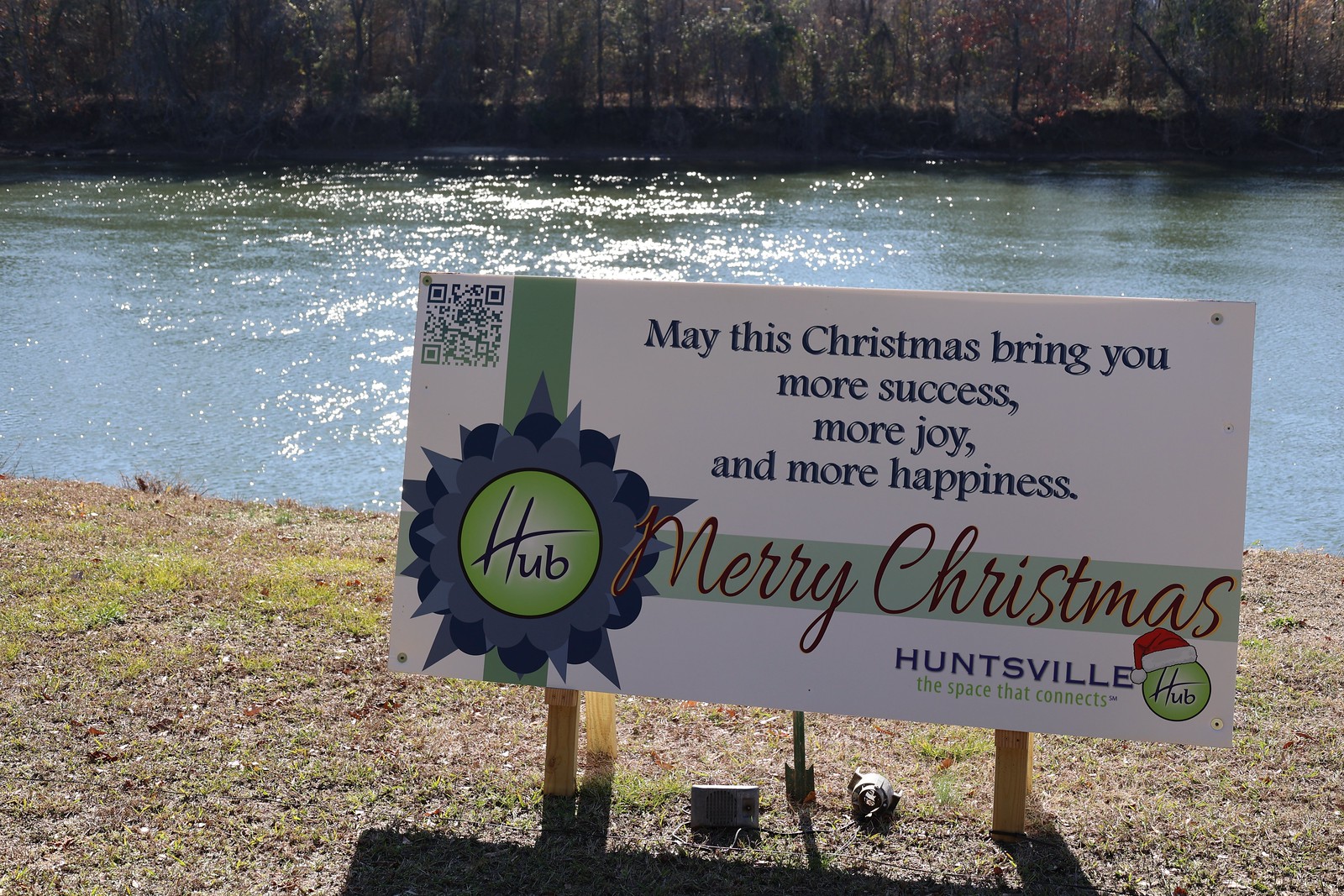The image captures a rectangular sign mounted on two wooden stakes planted in sparse, grassy ground by a river. The top of the image shows an embankment lined with trees, with the bluish-green river visible just below it. In the bottom portion, sparse grass is noticeable.

The sign itself is a long, white rectangle that is wider than it is tall. The upper section of the sign features a message in blue text that reads, "May this Christmas bring you more success, more joy, and more happiness." Just below this message, the phrase "Merry Christmas" is written in red cursive script spanning almost the entire width of the sign. To the left side of the sign, there's a festive design: a green ribbon running vertically, interwoven with another ribbon horizontally, forming a medallion-like structure with blue and green shades resembling a bow. Within this bow is the word "HUB" in black.

The lower section of the sign includes additional text. On the right side, the word "Huntsville" is written in blue, and below it, in green, it says, "the space that connects." Adjacent to this, there is another green circle containing the word "HUB" with a Santa hat on top.

In summary, the sign is a festive holiday greeting, blending Christmas wishes with local branding and set against a tranquil riverside background.